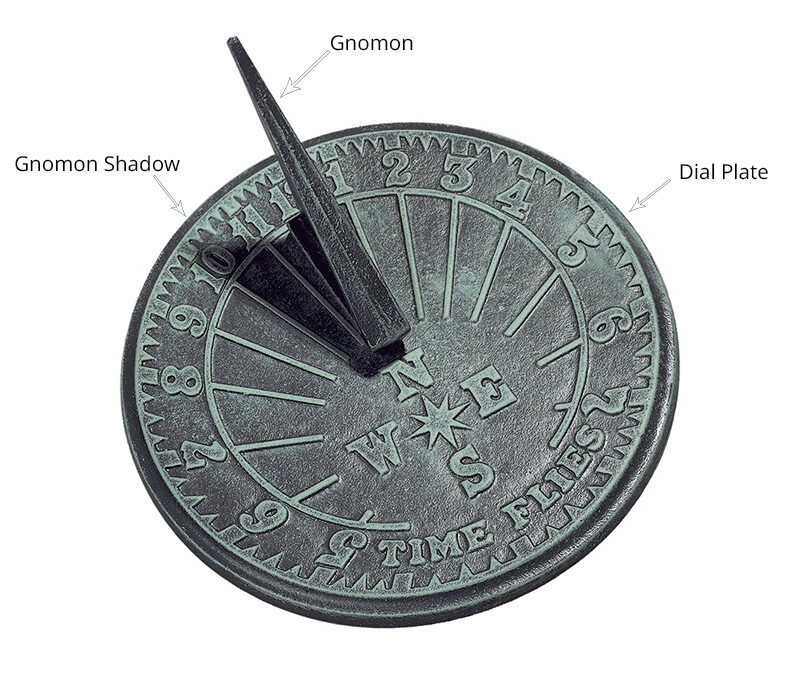This photo captures a detailed image of a circular, dark gray sundial tinged with a greenish copper hue. The sundial features a metallic surface and is inscribed with numbers, albeit in an unconventional manner—1 through 7 on the right half and 5 through 12 on the left half, arranged around the circle. At the base of the sundial is the phrase "Time Flies." Key components of the sundial are identified with labels: the "gnomon," which stands upright and casts a "gnomon shadow," and the "dial plate" that forms the main body. Cardinal directions—north, east, south, and west—are marked, enhancing the navigational aspect of the device.